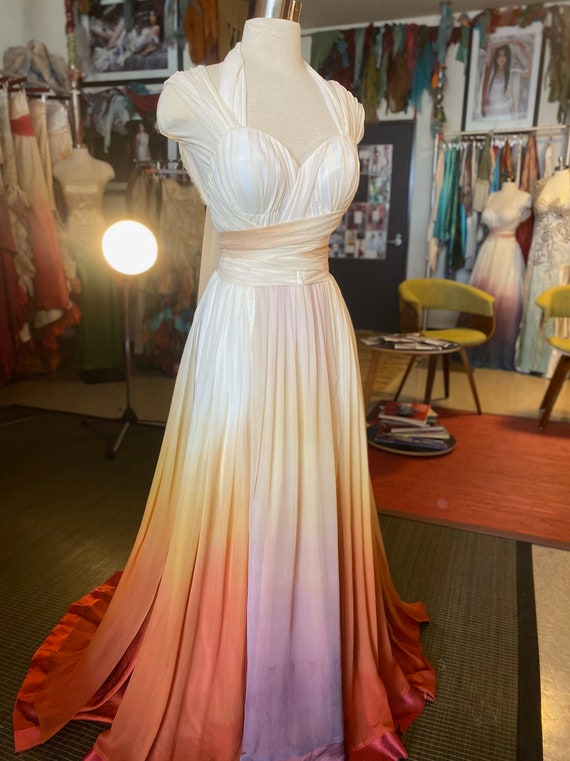The photograph captures a detailed scene inside a vintage dressmaking shop. The focal point of the image is a headless, armless mannequin adorned in an elegant gown. The dress is predominantly white at the top, featuring a sweetheart neckline and a cap sleeve that wraps around the neck and waist with a splash of color. As it flows down, the gown transitions into purple and vibrant orange hues, finishing with a pinkish-red at the bottom where it broadens out. Surrounding the mannequin, the shop appears dimly lit with a 1940s aesthetic, enhanced by a dusky ambiance. To the right, more dresses hang on racks and additional mannequins showcase a variety of formal, old-fashioned gowns. Portraits of women decorate the walls in both the upper left and right of the frame. A circular floor light is visible, casting a bright shine towards the scene, and a black floor rug anchors the setting. This image beautifully captures the timeless elegance and intricate detailing of vintage dressmaking.